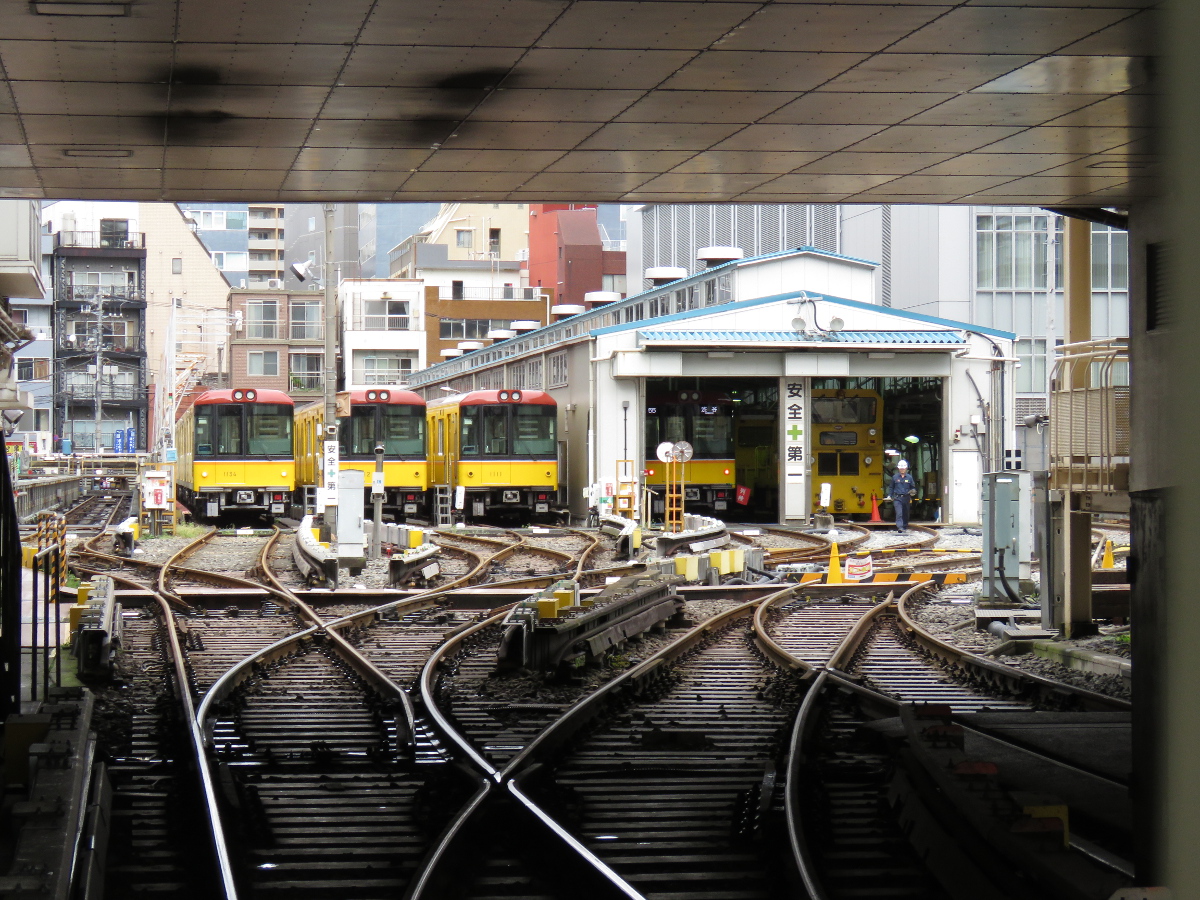The photograph vividly captures a bustling train yard within a cityscape, featuring a complex network of train tracks that converge from the foreground and lead towards the background. At the immediate bottom, train tracks twist and turn under a reflective, tiled ceiling which marks the covered area of the yard. Beyond this covered section, the scene opens up to reveal several lined-up trains.  

Five train cars dominate the middle ground, three of which display a striking yellow and red color scheme: yellow bodies with red rooftops. These trains are parked outdoors, slightly out of focus but still discernible. Two additional trains, including one with a distinct black and yellow appearance and lit interior, rest within a garage-like structure visible to the right. The other garage-train has a traffic cone and person in blue coveralls and a white hard hat nearby, indicating it is currently not in operation.

Further enhancing the urban backdrop, residential and industrial buildings in varied colors, sizes, and arrangements frame the train yard, lending a sense of a densely built-up area. Notably, some of the buildings bear indistinct Asian script, suggesting the location might be in an Asian country. The sky remains unseen, cloaked by the surrounding architecture, contributing to a grayish tone that permeates the scene. This richly detailed yard underscores both the vibrant functionality and the urban integration of the city's transit infrastructure.